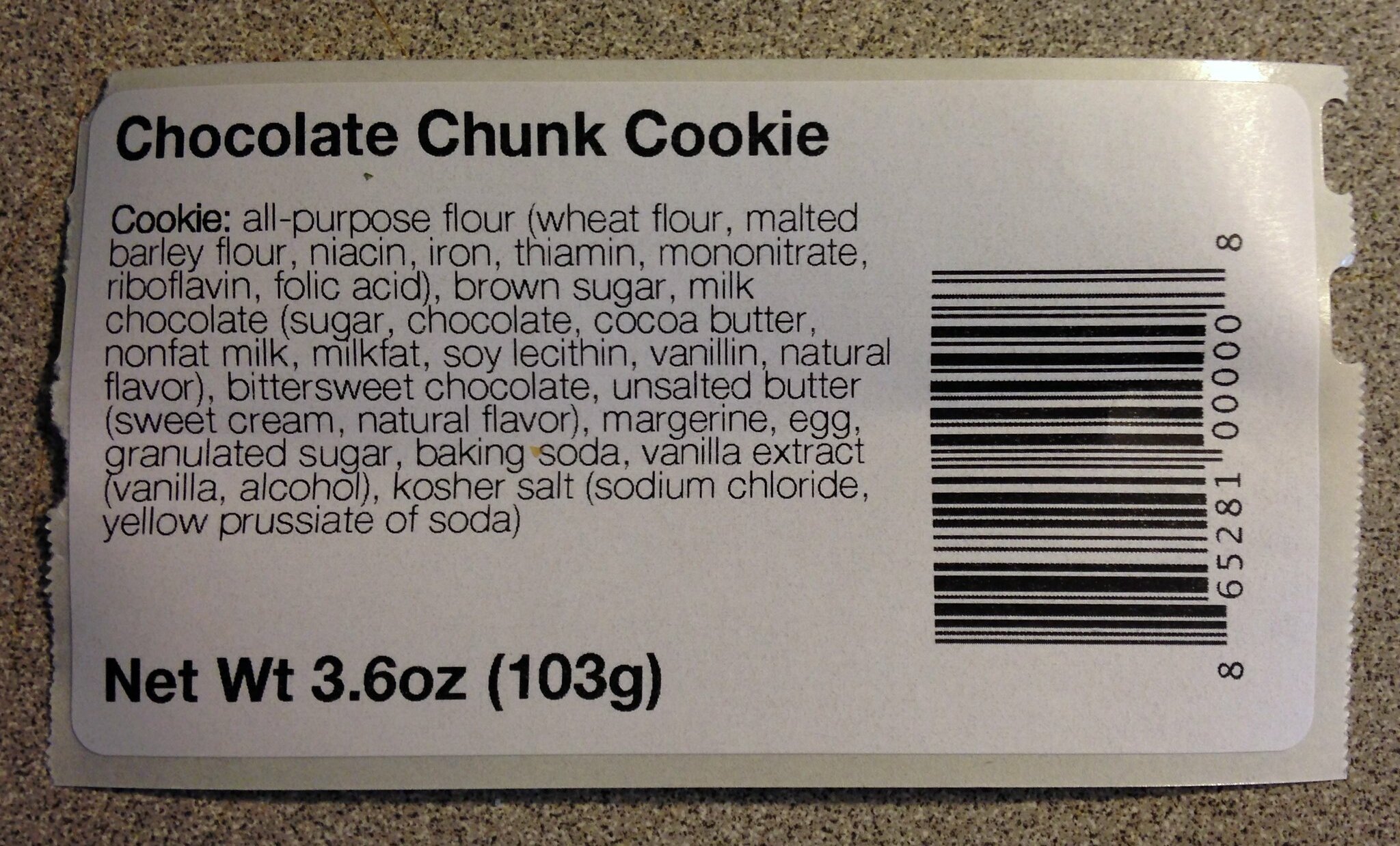The image depicts a detailed label for a chocolate chunk cookie, adhering to a wax paper background and placed on a multi-colored marble or granite countertop. The label itself is white with black text. Bold and prominent, "Chocolate Chunk Cookie" is displayed at the top, followed by smaller subtext listing the ingredients: all-purpose flour (wheat flour, malted barley flour, niacin, iron, thiamin mononitrate, riboflavin, folic acid), brown sugar, milk chocolate (sugar, chocolate, cocoa butter, nonfat milk, milk fat, soy lecithin, vanillin, natural flavor), bittersweet chocolate, unsalted butter (sweet cream, natural flavor), margarine (misspelled with an 'e'), egg, granulated sugar, baking soda, vanilla extract (vanilla, alcohol), and kosher salt. The bottom of the label notes a net weight of 3.6 ounces (103 grams). On the right side, a vertically-oriented barcode numbered 865-281-00008 completes the label's details.